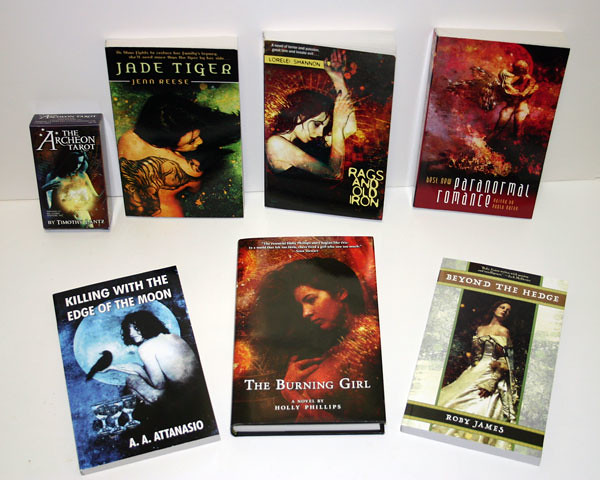The image depicts a collection of seven books arranged on a white surface against a white wall, creating a minimalistic and nondescript backdrop. Four of the books are standing upright, while three are lying flat. The standing books include titles such as "The Archer on Tarot," which appears more like a box, possibly a deck of cards, "Jade Tiger" by Jean Rees, "Rags and Old Iron," and "Paranormal Romance." The three books lying down are "Killing with the Edge of the Moon," "The Burning Girl," and "Beyond the Hedge." Each book features cover art primarily depicting women with long hair, either looking down or as portrait subjects. Despite variations in themes—ranging from fantasy romance to historical romance—the cover art connects them with a cohesive style. The overall composition offers a unique and striking visual, blending elements of fantasy and a hint of horror.